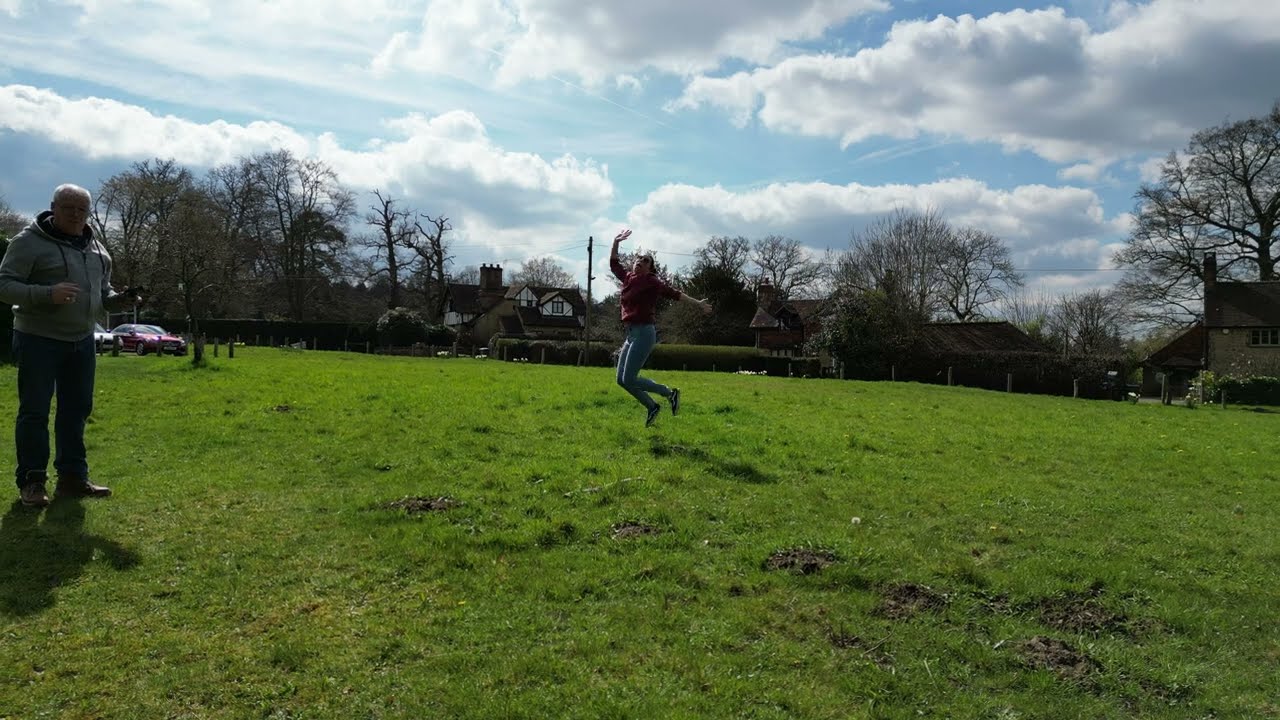This horizontally aligned rectangular photograph captures a lively daytime scene in a vast grassy field. On the left-hand side stands an older man with short gray hair, wearing glasses, a gray zippered hoodie, jeans, and boots. His face remains mostly in shadow as he stares directly at the camera. Centered in the image, a woman in a red long-sleeved shirt and blue jeans is caught mid-jump, her right arm raised high and the left extended behind her, creating a dynamic and playful pose. She accessorizes with sunglasses and tennis shoes, her expression conveying a sense of joy and spontaneity. The background features a row of houses, some two-story, interspersed with trees that have few leaves, and a fence lined with green hedges. Cars are parked behind the man to the left, adding depth to the setting. The sky above is a mix of blue and fluffy clouds with gray undersides, illuminated by sunlight from the upper left corner, offering a picturesque backdrop to this carefree moment.